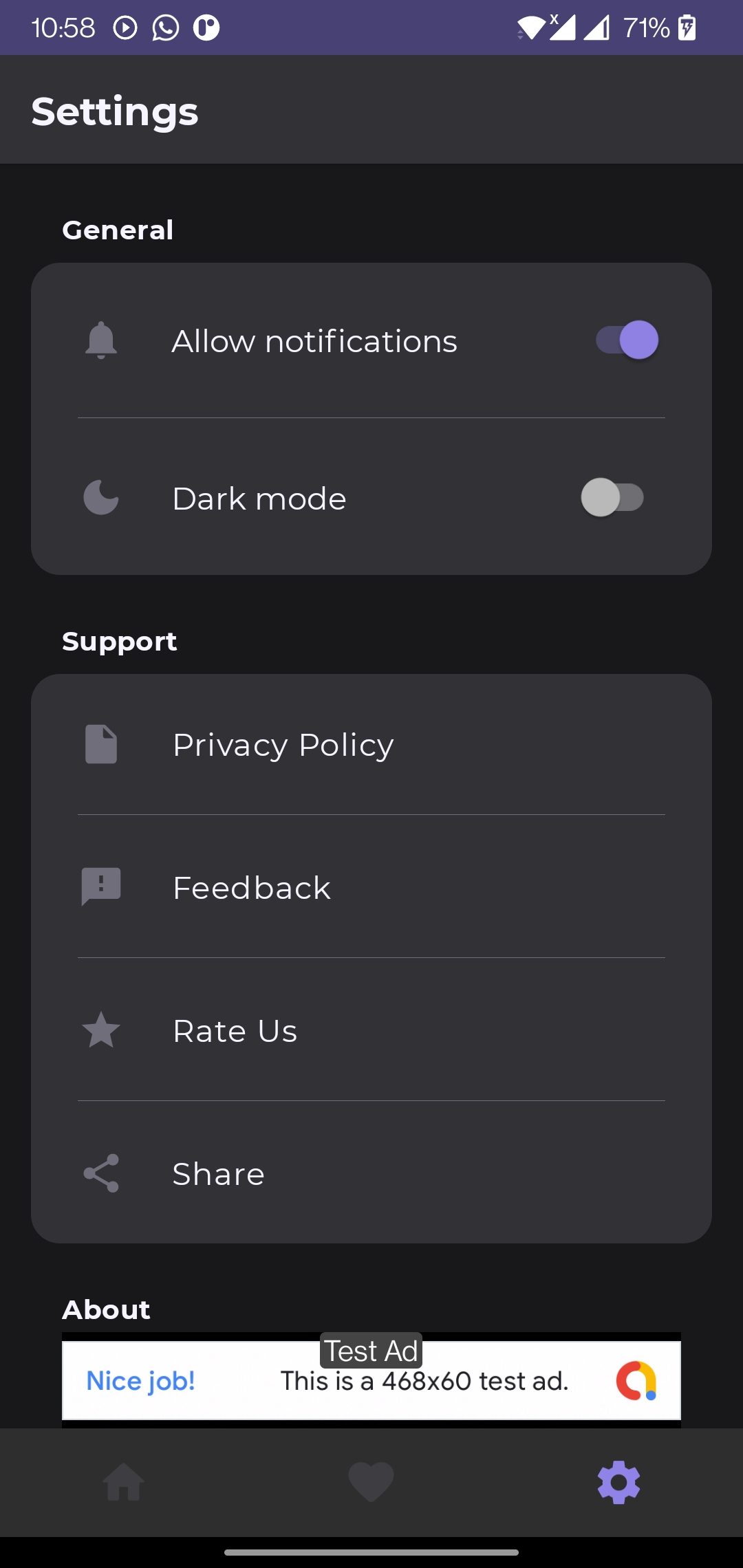This image is a screenshot of a mobile application interface featuring advertisements. 

At the very top, there is a narrow, purple bar stretching across the width of the image, displaying phone UI icons in white. From left to right, the icons include the time "10:58", a circular symbol with a triangle inside, a WhatsApp icon, and a purple "R" inside a white circle. Following these icons, on the top right, are the Wi-Fi connection symbol and the signal strength indicators for two SIM cards—the first signal indicator is at full strength while the second is almost full. Beside these is the battery icon showing 71% charge and is depicted vertically.

Below this purple bar, there is a dark gray section with white text aligned to the left, featuring bold, sans-serif, capitalized heading text that reads "Settings". 

The main section of the app follows, set against a black background. The first heading, "General", is in white text. Under this heading, there are two gray, rounded-edge sections. The first section is labeled "Allow Notifications", which has a notification symbol on the left and is toggled on. The next section is the "Dark Mode" option, featuring a moon icon on the left and is toggled off.

A space separates these sections from another heading, "Support", also in white text. Below this heading is a second gray, rounded-edge section containing four rows: "Privacy Policy", "Feedback", "Rate Us", and "Share". 

The bottommost part of the main section has the heading "About" followed by an advertisement that reads, "Nice job. This is a 468 by 60 test ad", with "test ad" prominently displayed.

Finally, the bottom part of the image shows additional phone UI elements. These include a row of icons starting with the home button on the left, a heart icon in the middle, and a settings icon on the bottom right. The settings icon matches the purple hue seen at the top of the image, though possibly lighter. Below these icons is a thin gray line that spans about half the width of the image, set against a black bar background.